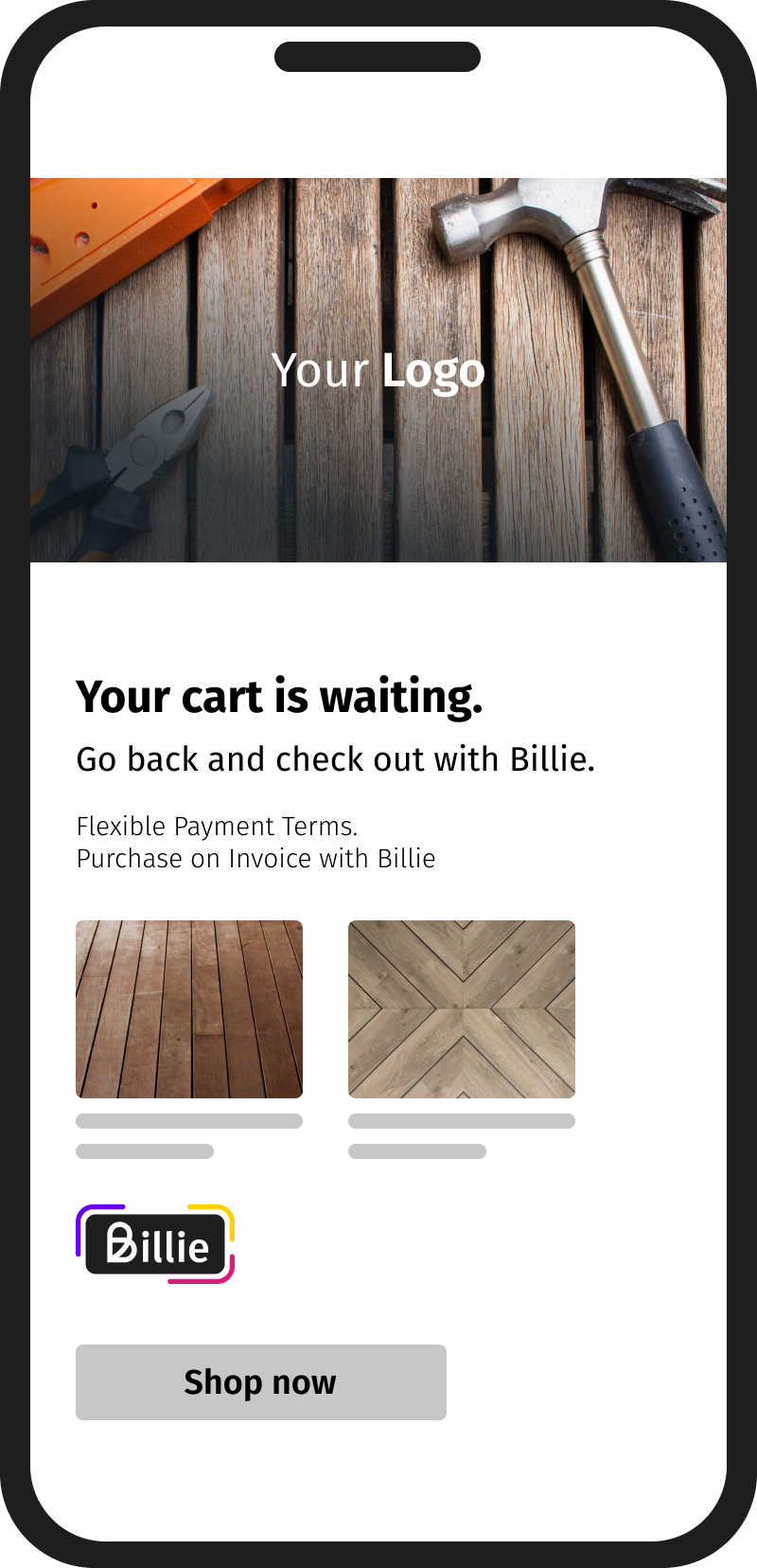The image is a screenshot designed to look like it's displayed on a smartphone. It features a white background with a prominent photograph at the top, showcasing a selection of hand tools, including a hammer, a pair of pliers, and an orange leveler, all resting on a wooden platform or wooden planks. In the center of this photograph, white text displays a logo.

Beneath the image, bold dark text on the white background reads, "Your card is waiting." Following this, smaller text instructs, "Go back and check out with Billy." 

Below these phrases, two lines of text state, "Flexible payment terms," and "Purchase on invoice with Billy."

Further down are two images depicting wooden flooring. The first image shows light brown, narrow planks aligned vertically, while the second image features a floor with an intricate X-type design in light beige with a stain effect.

At the bottom, there is a button with a logo, black with white text reading 'Billy,' and bordered in vibrant colors purple, yellow, and magenta. Below that is a larger greyed-out button with the text, "Shop now."